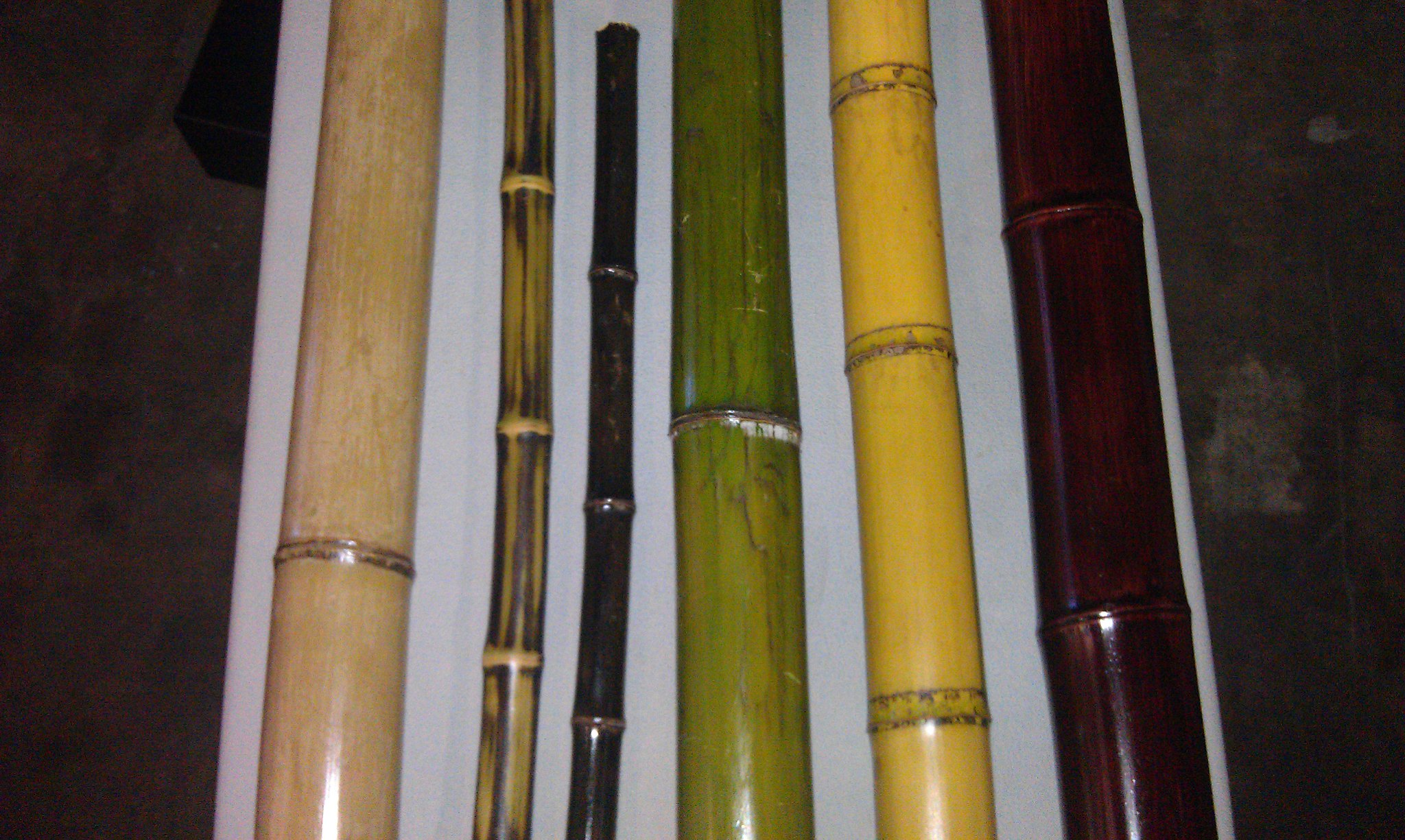This color photograph features a sharply detailed close-up of six bamboo reeds arranged side by side on a white background, which could be a shelf or piece of cloth. The image is framed by a predominantly dark brown-black background with smudges and shadows at the far sides, creating a vivid contrast with the lighter center. Each reed has distinguishing characteristics:

- **The first reed on the left** is light brown, almost tan, and is one of the thickest. It has a round metal section towards its bottom and consists of two divisions.
- **The second reed** is thin and striped with green and black, featuring three metal parts around it.
- **The third reed** is extremely thin and blackish-brown in color, also divided into four sections by metal rings.
- **The fourth reed** is slightly thinner than the first and is light and dark green mixed, marked by a metal ring in the middle, and composed of two sections.
- **The fifth reed** is yellowish with three darker rings, divided into four sections.
- **The sixth and final reed** is dark reddish-brown, thick like the first one, and split into three metal-ringed sections.

The central focus and bright illumination highlight the intricate details and textures of the reeds, while the darker periphery maintains the viewer's attention on the central objects, contributing to the overall composition's aesthetic.